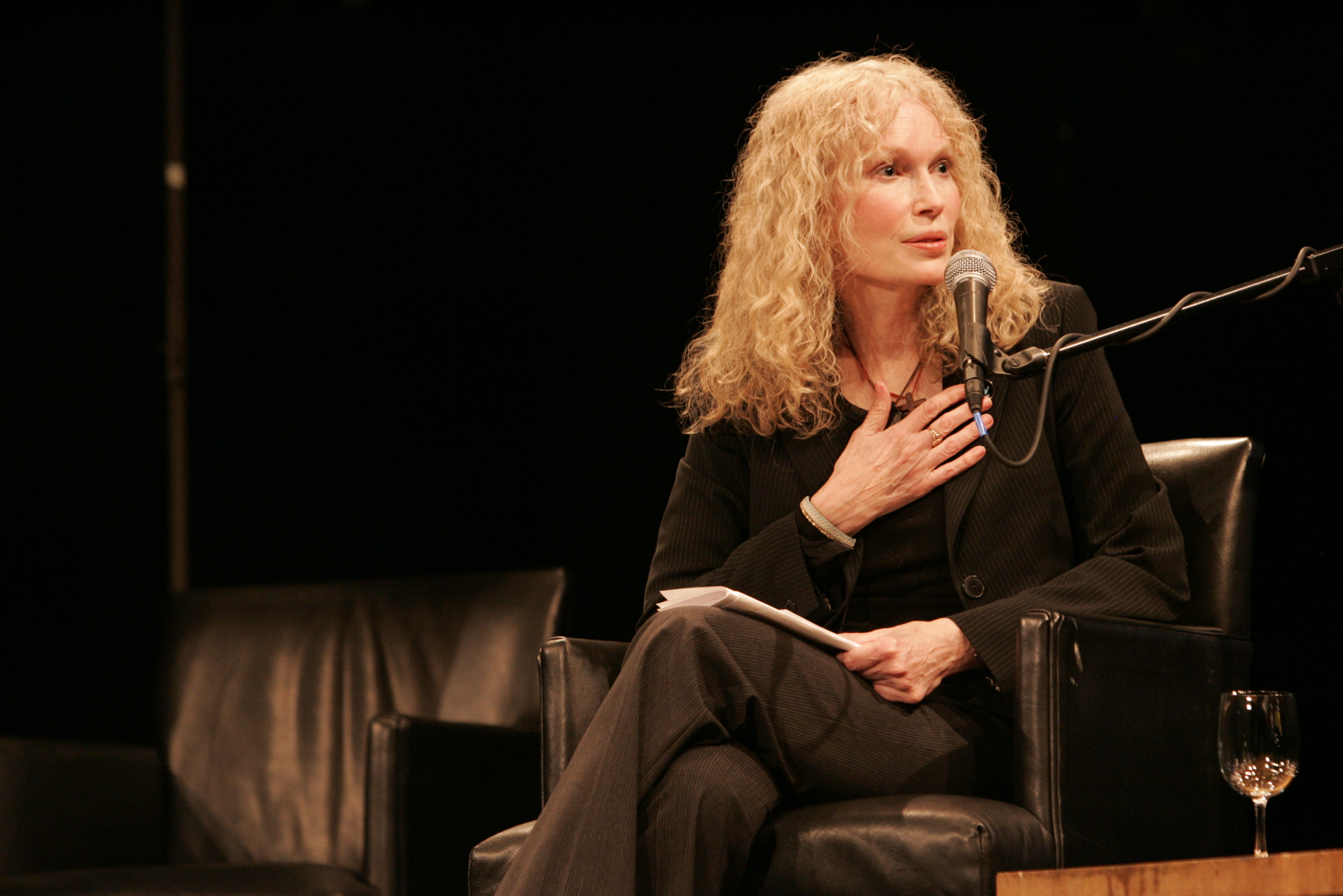In this photograph, a woman in her 40s or 50s is captured speaking into a microphone at an event. She is seated in a low black leather chair, with another identical, but empty, chair to her left. The backdrop is entirely black, providing a stark contrast to the scene. The woman has shoulder-length, curly blonde hair and is wearing an unbuttoned black pantsuit with a black shirt underneath. Her legs are crossed, and one hand is resting on a set of folded papers on her lap while the other hand, adorned with a bracelet, is placed over her heart. A necklace with a cross hangs around her neck. She gazes to the right, with her mouth slightly open as she speaks. To her right, a table corner is visible with a wine glass that appears to contain a light brownish liquid.